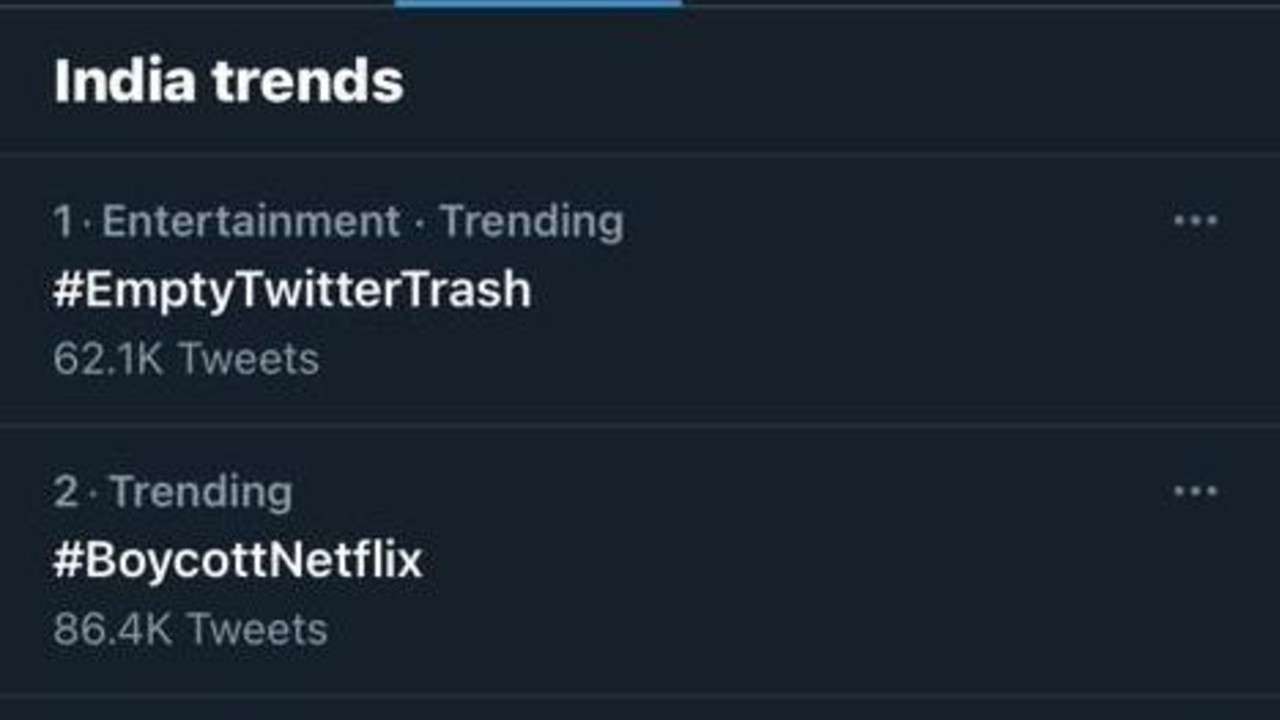Here is the cleaned-up and detailed caption:

---

This image is a screenshot showcasing a portion of a Twitter interface, specifically highlighting trending topics in India prior to the platform's rebranding as X. The background hue is a subdued black. At the top of the screenshot, the title "India Trends" is prominently displayed in bold white font. Immediately beneath the title, a faint horizontal white line creates a subtle division.

The first trend listed is labeled "1. entertainment.trending" with the associated hashtag "#EmptyTwitterTrash" highlighted below, which has accumulated 62.1K tweets. Positioned in the upper right corner adjacent to this entry are three horizontal white dots, indicative of additional options.

Following this, the second trend appears, simply marked as "2. trending" with the hashtag "#BoycottNetflix" mentioned below, showing a higher tweet count of 86.4K tweets. Similarly, three horizontal white dots are aligned to the right of this entry, continuing the option menu interface.

Another faint horizontal white line is depicted beneath this second trend, partially obscuring what presumably continues as a list of trending topics in India on Twitter, though the bottom-most entries are cut off in this screenshot. 

This detailed capture provides an insight into the trending discussions among Indian Twitter users at the time.

---